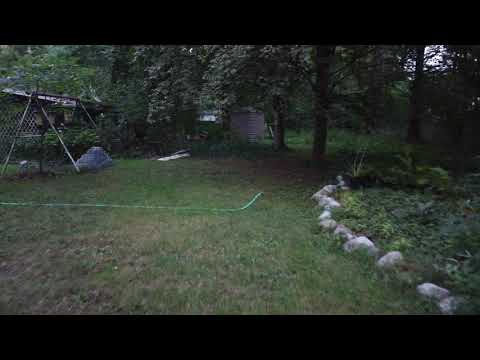This color photograph captures a realistic view of a backyard in landscape orientation. The grassy yard features a short, native grass that is patchy with some dry spots. A green garden hose runs across the center of the yard, veering upwards and away into the distance. At the top left of the image, an older model gray metal swing set, reminiscent of a teepee style, stands partially obscured. It's unclear whether the swings are still attached. Toward the back of the yard, a row of trees conceals several outbuildings or sheds, along with potential wood piles. On the right side of the yard, there is a garden area or flower bed framed with large decorative gray rocks that curve onto the lawn. The photograph itself measures five inches wide by four inches tall, with a distinctive black strip running horizontally along both the top and bottom edges.